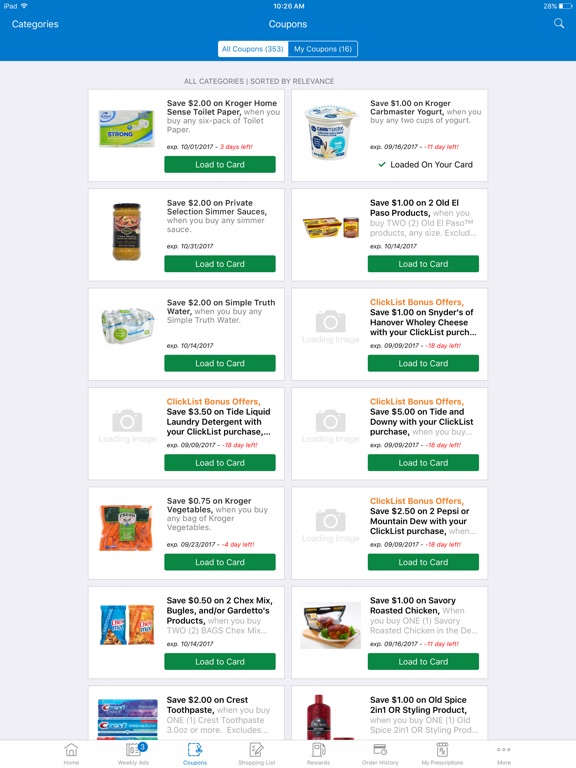A detailed and cleaned-up caption for the image:

---

The screenshot, captured from an iPad at 10:26 a.m. with 28% battery and Wi-Fi enabled, depicts a coupon webpage interface. There is a distinctive blue navigation bar at the top of the page. On the left side, white text lists categories, followed by a centered "Coupons" section, and a search icon located on the far right.

The main section of the page highlights two main coupon categories: "All Coupons" in blue text within a white box displaying 353 available coupons, and "My Coupons" also in blue text within a white box showing 16 selected coupons. The coupons are sorted by relevance, with a variety of products listed, each accompanied by a small descriptive box. These boxes detail the item, the discount offered, and feature a green "Load to Card" button for easy application.

Examples of available coupons include:
- "$32 on Simple Truth Water"
- "Save 75% on Kroger Vegetables" with a four-day expiration
- "Save 50 cents on two Chex Mix, Bugles, and/or Gardetto's products."

At the bottom of the page, a navigation menu provides access to several sections such as Home, Weekly Ads (noting three available ads), FBC Coupons, My Shopping List, Rewards, Order History, My Prescriptions, and a More options button. This comprehensive interface allows users to quickly and efficiently find and apply coupons to their loyalty cards.